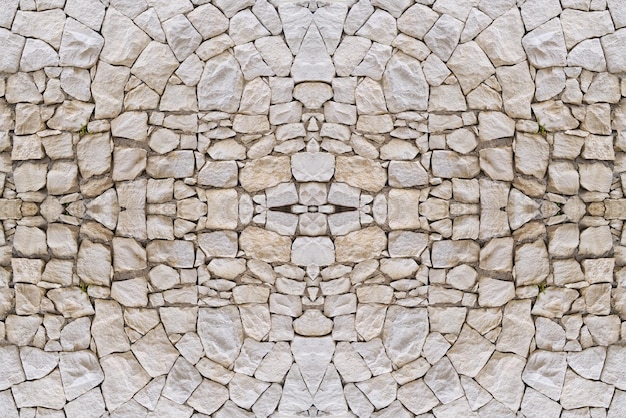This image captures an intricately designed abstract pattern made from white limestone rocks. The composition, which could be part of a wall or a floor, showcases a symmetrical and geometrically structured design. At the center, two larger squares are divided by slender pieces into two smaller squares, leading to three larger squares at the top. Interspersed small triangle pieces and a heart-shaped rock culminate into a large triangle, adding complexity to the pattern. The stones' colors vary, with light sandy tones at the top and bottom and a darker brown hue at the center. The entire design stretches to the edges of the image, emphasizing the meticulous arrangement and harmony of the stonework.